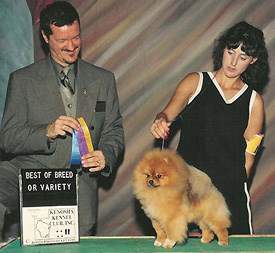In a warmly lit room with wood-paneled walls arranged diagonally, a well-groomed Pomeranian dog stands proudly on a green table, its long brown fur meticulously fluffed. The scene is set at a dog show, indicated by a sign that reads "Best of Breed or Variety," though the smaller text below is difficult to decipher. On the left side, a man dressed in a sharp gray suit with a matching tie and sporting a mustache smiles down at the dog, holding three award ribbons in his hands, ready to present an accolade. On the right, a slender woman, possibly in her early 20s, stands behind the dog. She wears a black sleeveless dress with white trim and has medium-length curly hair. The woman, who appears to be the dog’s handler, gently holds a short leash, her demeanor calm and proud as they await the award for their Pomeranian’s exceptional performance.